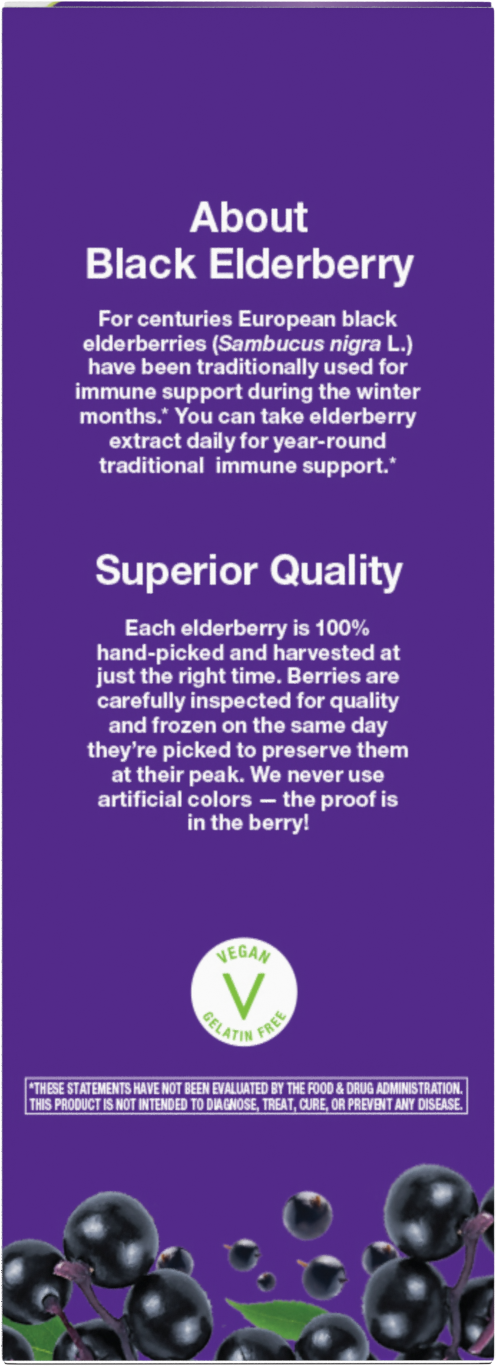This is a detailed description of an elongated, rectangular print ad or possibly a section of a box with a solid purple background. The design resembles the shape of a bookmark, making it much taller than it is wide. At the bottom of the image, there is a small photo depicting dark black elderberries accompanied by a few leaves, which resemble deeply purple-colored blueberries.

In the center of the image, there are two white text blocks providing detailed information about the product. The first text block discusses the traditional uses of European black elderberries (Sambucus nigra L.) for immune support, particularly during the winter months. It emphasizes that elderberry extract can be taken daily for year-round immune support. The second text block, labeled "Superior Quality," highlights the meticulous process involved in harvesting the elderberries. Each berry is 100% hand-picked at just the right time, carefully inspected for quality, and frozen on the same day to preserve their peak condition. The product boasts of never using artificial colors, summed up with the phrase "The proof is in the berry."

At the bottom of the image, there is a round white circle featuring a vegan certification logo and an FDA warning, adding authenticity and trustworthiness to the product. The circle also mentions "vegan guarantee" and "gluten-free," underscoring the product's suitability for various dietary preferences.